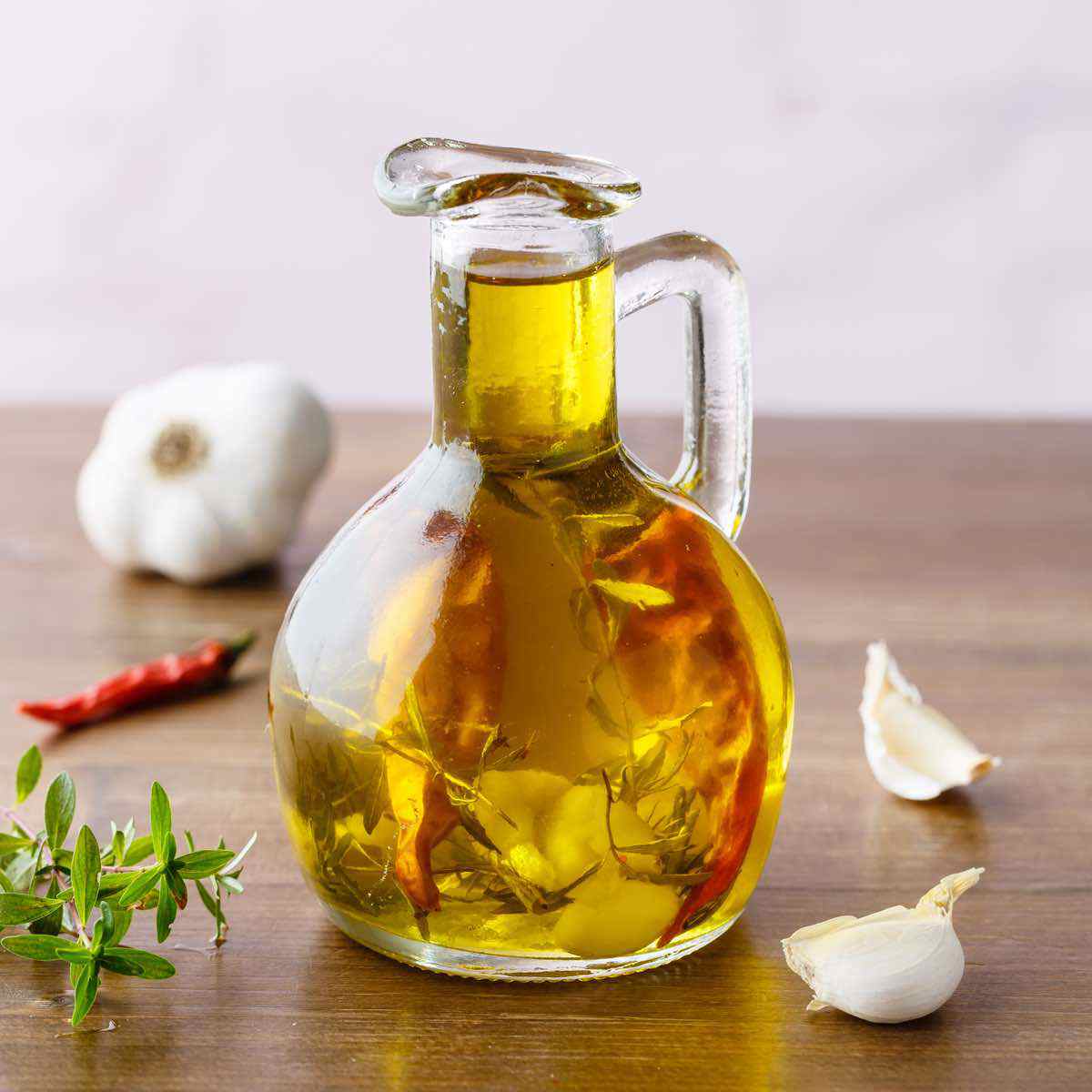The image showcases an elegant, clear glass decanter with a long neck and a handle, filled with what appears to be yellow olive oil. Inside the decanter, various spices are visible, including garlic cloves, green herbs, and a red pepper with a green tip. The decanter rests on a brown wooden table. Surrounding the decanter, there are several garlic cloves, some taken apart, a whole bulb of garlic, and a red pepper. The overall setup suggests that these items might be the same ingredients infused within the olive oil inside the decanter. The background of the image is plain white, keeping the focus on the decanter and its accompanying spices. The neck of the decanter is notably thinner than its body, and there is no lid on it.